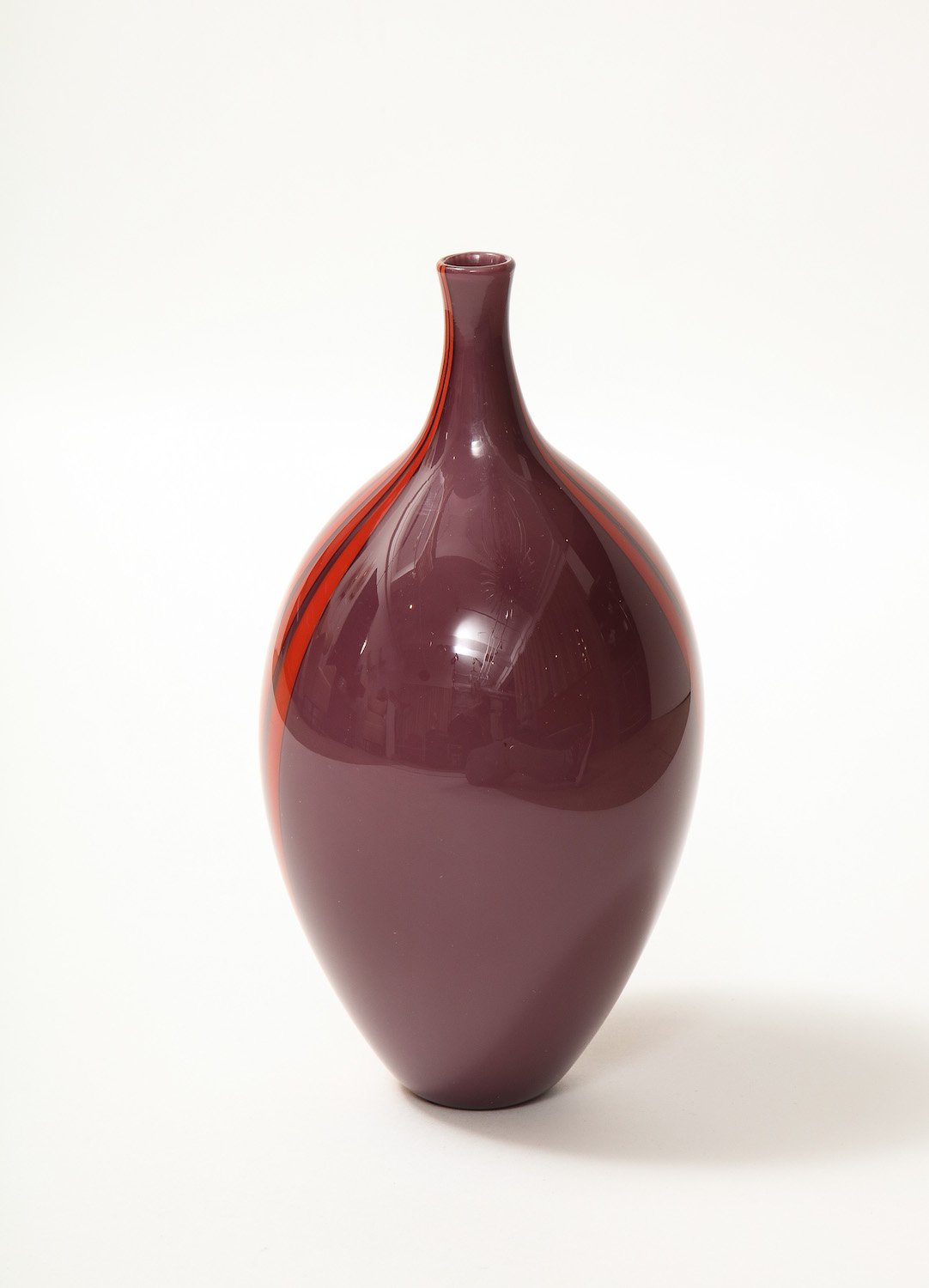The image displays a possibly antique ceramic vase, which might be for sale or serve as a sample piece. Set against a white background and placed on a white table, the vase casts a shadow extending towards the right of the picture. The vase itself is predominantly a light maroon or burgundy color and boasts a distinctive design. It features a narrow spout approximately 3 to 4 inches tall that broadens into a wide, rounded body, resembling a teardrop shape, before tapering slightly again at the bottom, though not as narrow as the spout. The vase is adorned with bright red or neon orange-red stripes on both sides, which extend from the top of the spout downwards, at least halfway along the vase, if not further. The vase's shiny surface reflects its surroundings, adding to its elegant appearance.